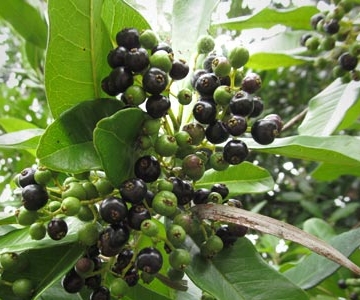This close-up, color photograph captures clusters of olives growing on a tree branch, taken outdoors during the day. The image, in landscape orientation, emphasizes the large green leaves and various clusters of small, spherical olives at the center. The olives, ranging in color from dark purple, almost black, to medium green, indicate different stages of ripeness. These olives, all roughly the same size, are attached to stems emanating from a central branch. Surrounding the olives, large, broad, oval-shaped leaves dominate, while a distinctive darker, palm-like leaf extends towards the bottom right corner. The background is intentionally blurred, with foliage and an additional cluster of olives slightly out of focus in the upper right, giving the scene depth. Notably, the image captures the intricate details, such as the indentations in the olives and the interplay of light creating a brighter patch towards the top center. The photograph employs a realistic style, emphasizing texture and natural beauty.